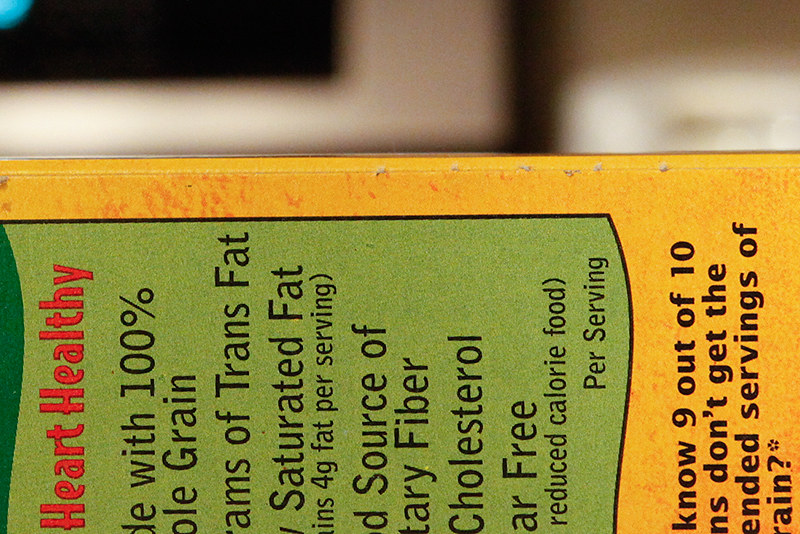The image is a landscape-oriented photograph of a partially visible food product box turned on its side, occupying the bottom three-quarters of the frame. The background is dark and blurry with what seems to be white angular shapes, possibly boxes, and a black computer screen with some blue elements. The box's primary color is a yellowy-orange with a prominent green text panel. Clear red text on the box states "heart healthy." Various other details can be discerned in black font, including "made with 100% whole grain," mentions of "grams of trans fat," "saturated fat," "4G fat per serving," "source of dietary fiber," "cholesterol-free," and "reduced calorie food per serving." Additionally, there is a note that reads, "9 out of 10 [NS] don't get the recommended servings of grain," with an asterisk marked by a flower symbol in superscript.